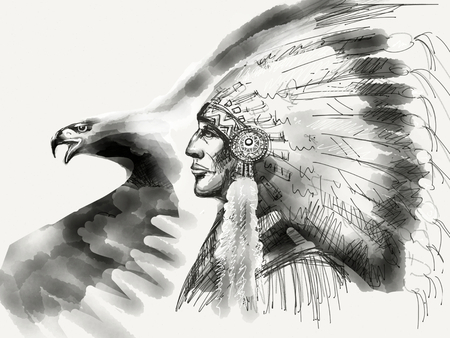This detailed drawing combines pencil and watercolor techniques to depict a Native American man, possibly a chief, in profile. His expression is stoic, enhanced by a prominent hooked nose and lips. He dons a traditional, elaborate feathered headdress complete with a beaded headband, a round medallion near his ear, and strands of smaller feathers hanging below. The feathers of the headdress rise in a wide fan behind him, displaying intricate detailing even amidst the abstract renderings. To the left of the man is the profile of an eagle with its beak open, depicted with striking accuracy. The eagle's wings are rendered abstractly, with one wing flowing off the page and the other extending over the man, creating an illusion that melds the two figures together. The eagle’s wings and parts of its body dissolve into splotches of watercolor, giving an impression of ethereal disintegration. The entire composition is monochromatic, employing shades of black and white to produce depth and shadow, with the watercolor bleeding into the sketch lines, adding a dramatic and haunting effect that unifies the man and the bird in a dynamic visual narrative.